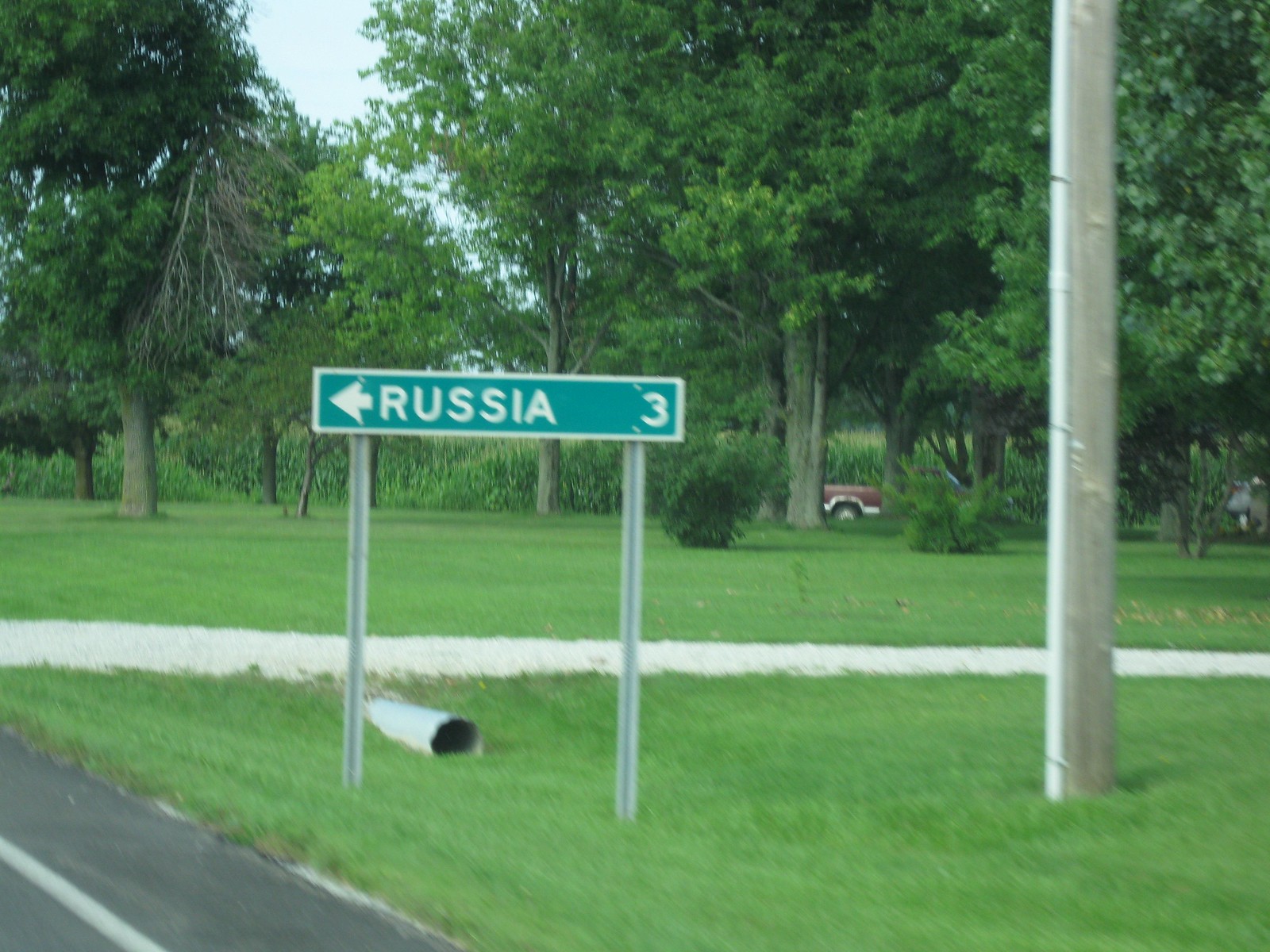In this outdoor photograph, captured from inside a vehicle, the foreground features a section of pavement with a white line marking its edge, adjacent to a grassy area. Dominating the scene is a narrow, green street sign mounted on two metal posts, displaying "Russia 3" along with a white arrow pointing left. The sign is bordered in white, adding to its visibility. Directly beneath the sign, a metal culvert or pipe extends beneath a dirt or gravel path running parallel to the sign. To the right, there's a utility pole amidst the grassy expanse. The backdrop showcases a cluster of deciduous trees, with a brown pickup truck partially visible, its rear end emerging from behind the foliage and blending into the natural setting.